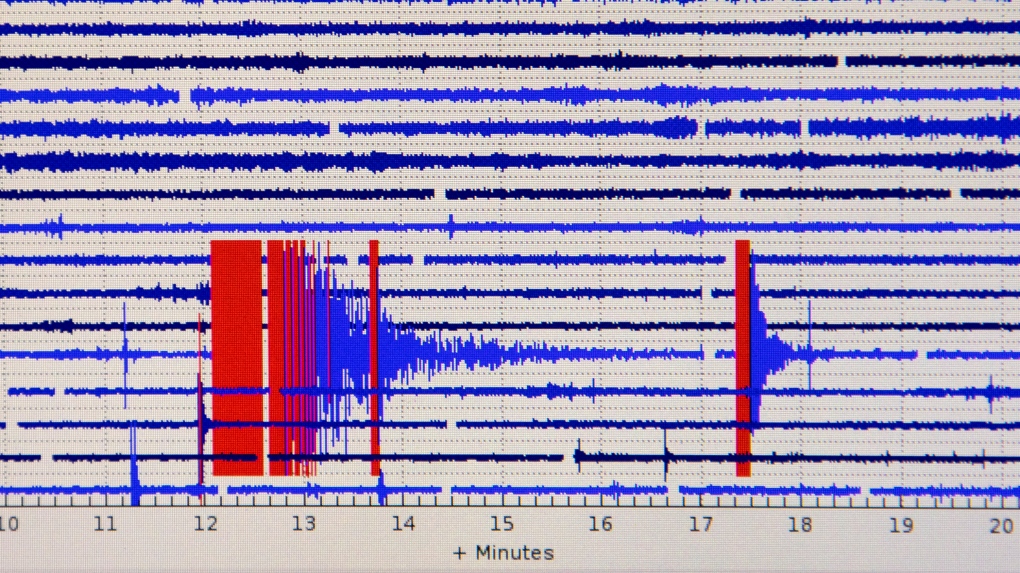The image depicts a detailed recording of different wavelengths, resembling outputs from a seismograph, lie detector, or echocardiogram. There are 15 horizontal blue lines, each representing various measurements. The intensity of these lines changes with the amplitude; the shorter wavelengths are depicted in darker blue, while the larger ones are a lighter blue. Notably, there are highlighted sections in red, particularly around the 12–14 and 17–18 minute marks, indicating significant activity recorded. The background and border are gray, with a time scale at the bottom ranging from 10 to 20 minutes, marked in a dark gray color with "plus minutes" labeled beneath it.